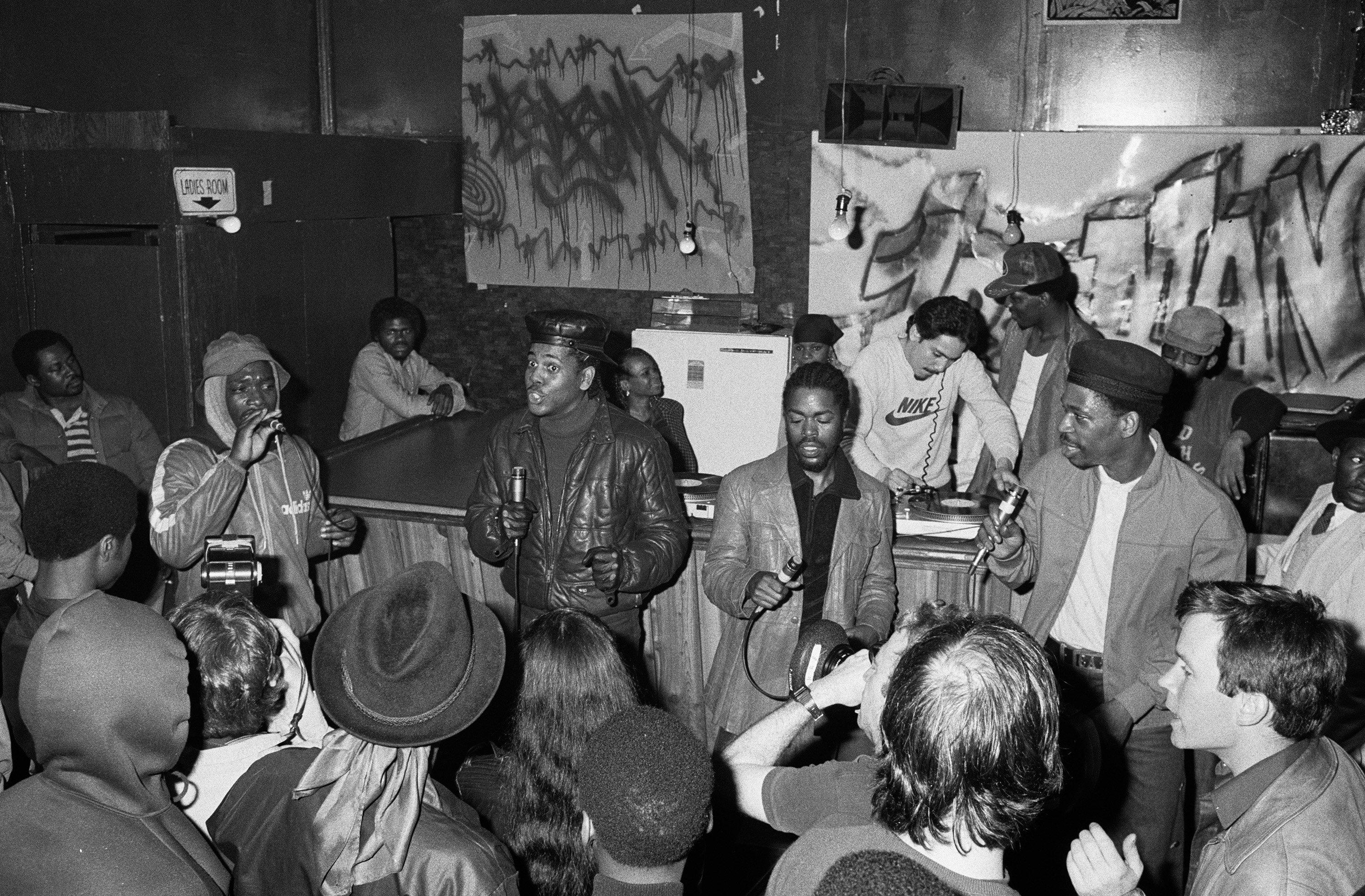The black-and-white flash photograph captures a vibrant and electrifying scene from a likely late 70s to mid-80s nightclub or concert atmosphere. At the forefront, four African American men are each passionately speaking into microphones, suggesting a live rap performance. They are dressed casually, consistent with the era's style. The crowd, inclusive of at least one white woman with long hair in the bottom left, is mostly turned away, intently watching the performers. The venue's decorations include large sheets adorned with graffiti art and a sign marked "Ladies Room" with an arrow pointing left, adding to the urban ambiance. A bare light bulb hangs from the ceiling, casting dynamic shadows. In the backdrop, a DJ in a white Nike sweater is skillfully spinning records on a turntable, anchoring the scene as an authentic representation of an early rap concert.